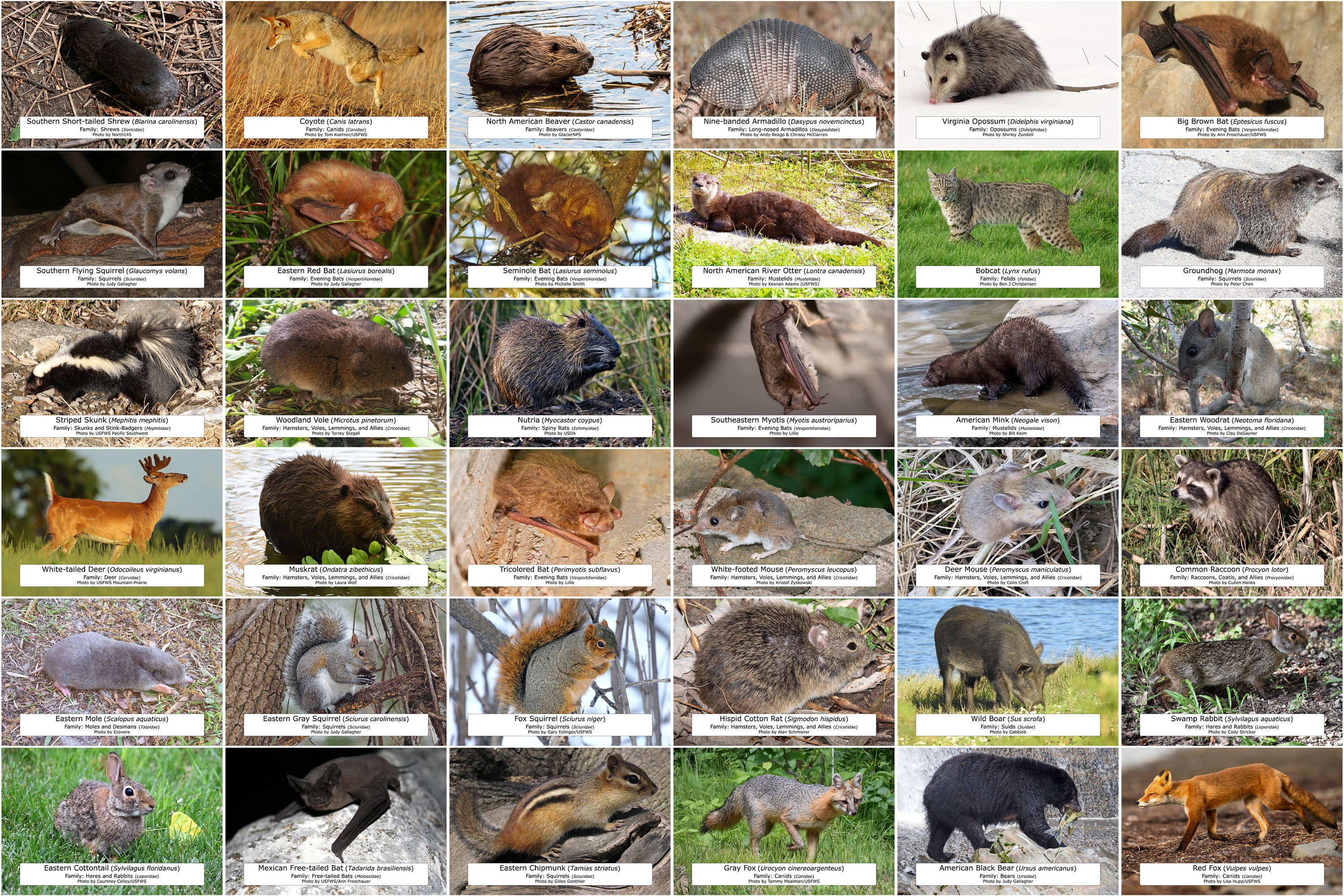This image is an educational composite graphic featuring 36 candid photographs of various North American woodland animals, organized in a 6x6 grid. Each photo is labeled with a small white text box that includes details such as the animal's name, its Latin name, family classification, and the photographer's credit, although these details are not readable in the image. The animals depicted span a broad array of species, including a beaver in the water, a coyote, an opossum, several types of bats, a leopard, various squirrels such as a red squirrel and a gray squirrel, a skunk, a raccoon, a white-tailed deer with antlers, different species of mice, foxes including a gray fox and a red fox, a rabbit, a bobcat, a wild boar, a black bear, an otter, a groundhog, an armadillo, a marmot, a flying squirrel, a wolverine, a mountain lion, an Eastern Chipmunk, an Eastern Cottontail Rabbit, and a Mexican Freetail Bat. All the animals are photographed in their natural habitats, providing a comprehensive overview of North American mammalian wildlife.